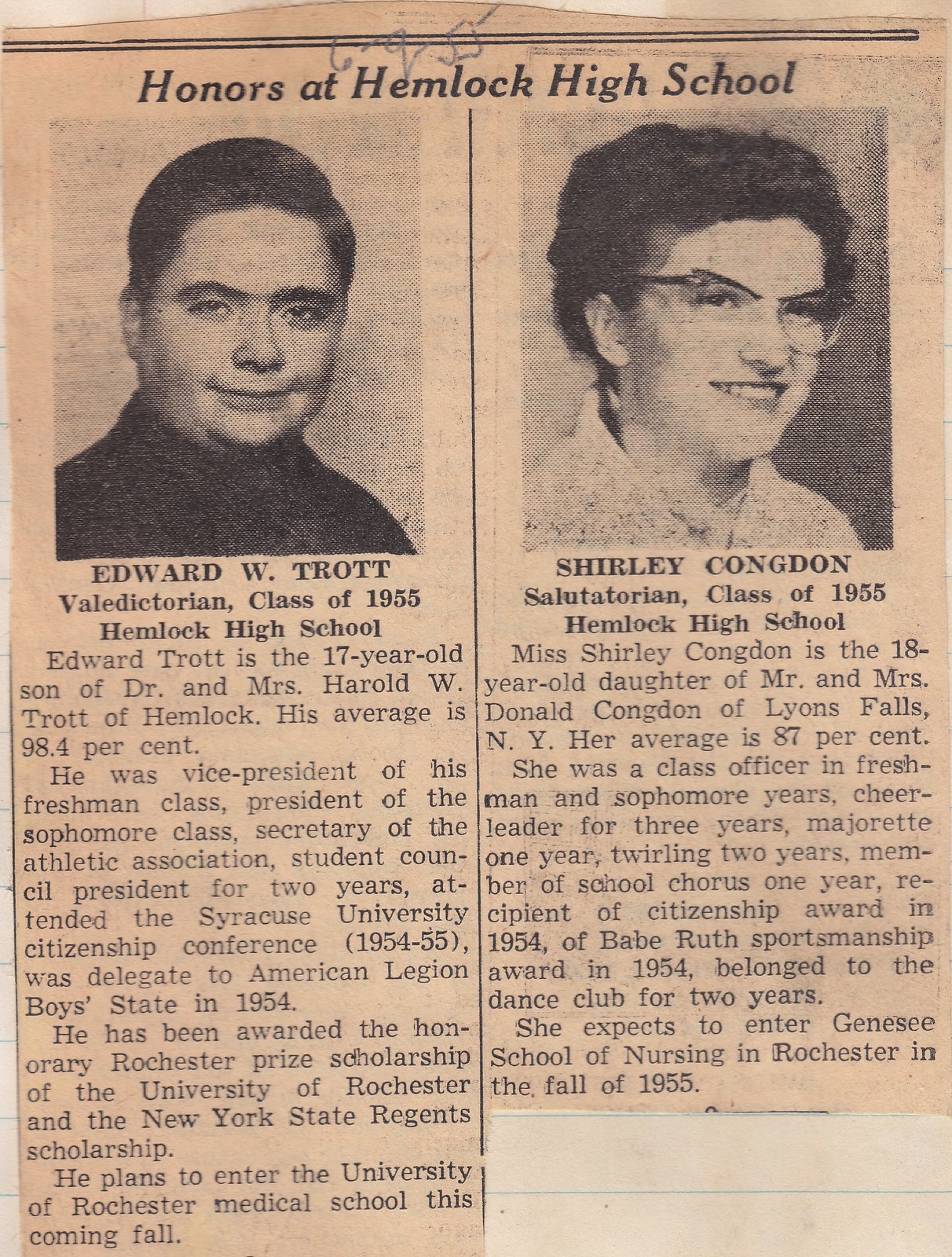The scanned image is a newspaper article titled "Honors at Hemlock High School," prominently displayed at the top in bold black text. Handwriting above the title reads "6955." The article is divided into two sections by a solid black line. The section on the left features a photo of a young man, identified as Edward W. Trott, the valedictorian of Hemlock High School's class of 1955. Under his name, it details that Edward is the 17-year-old son of Dr. and Mrs. Harold W. Trott of Hemlock. His academic average is 98.4%. Edward held several leadership roles, including vice president of his freshman class, president of the sophomore class, secretary of the Athletic Association, and president of the student council for two years. He attended the Syracuse University Citizenship Conference (1954-55) and was a delegate to the American Legion Boys State in 1954. He has been awarded the honorary Rochester Prize scholarship and the New York State Regents Scholarship. Edward plans to attend the University of Rochester Medical School in the fall.

The section on the right displays a photo of a smiling young woman with glasses, identified as Shirley Congdon, the salutatorian of Hemlock High School's class of 1955. Shirley is the 18-year-old daughter of Mr. and Mrs. Donald Congdon of Lyons Falls, New York. She has an academic average of 87%. Shirley was a class officer in her freshman and sophomore years, a cheerleader for three years, a majorette for one year, and involved in toiling for two years. She was a member of the school chorus for one year, received the citizenship award in 1954, and the Beirut sportsmanship award in 1954. She also participated in the dance club for two years and plans to attend the Gene C. School of Nursing in Rochester in fall 1955.